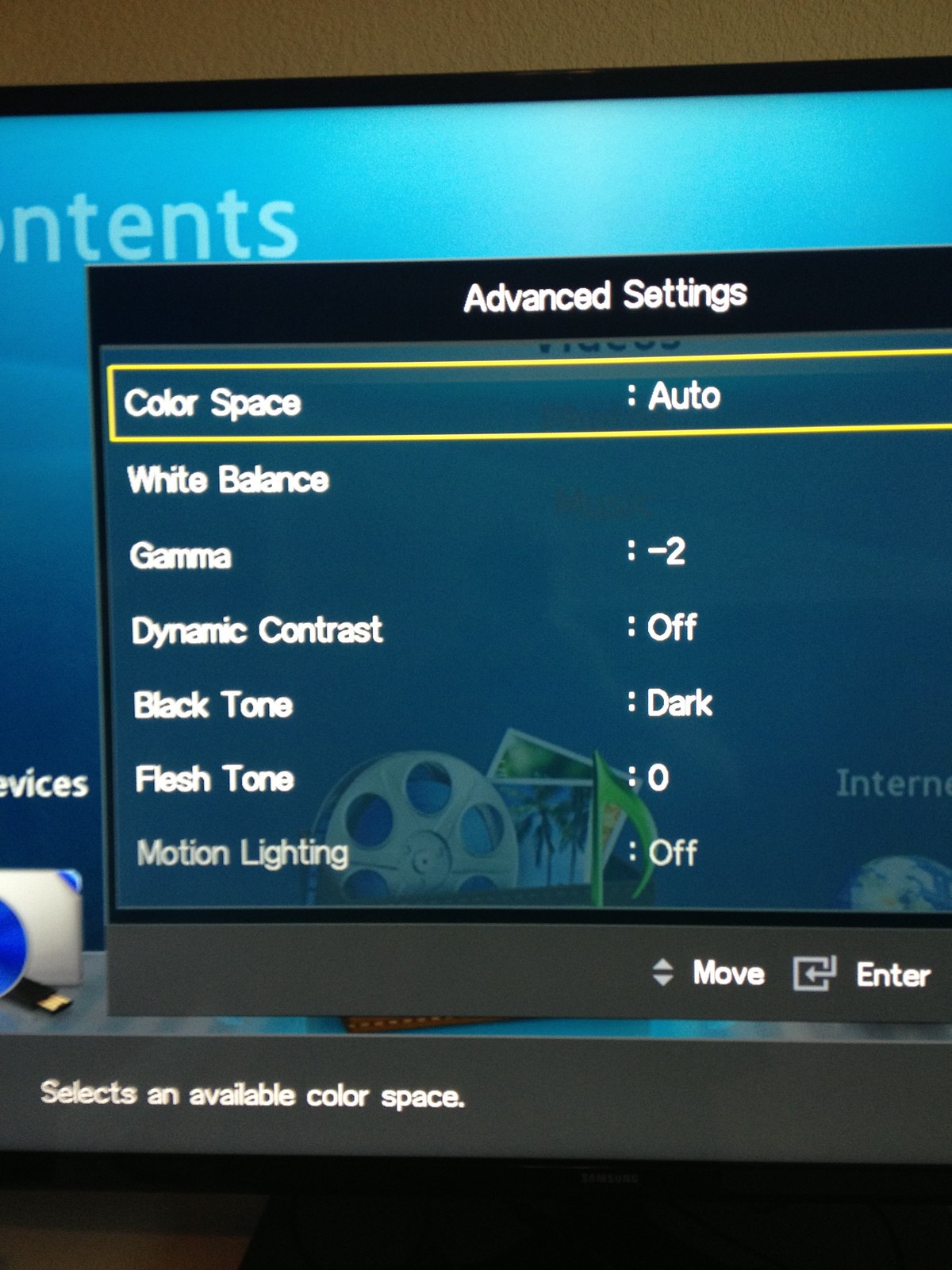This image captures the advanced settings menu on a television screen, indicating an adjustment or calibration process. The backdrop features a bluish gradient with various option icons. The settings include: color space set to "auto," white balance, gamma adjusted to "-2," dynamic contrast turned "off," black tone set to "dark," flesh tone at "0," and motion lighting disabled, indicated by its grayed-out appearance. The screen also displays the message "Select an available color space." The presence of familiar screen elements suggests this is part of routine setup or optimization for a clearer display.